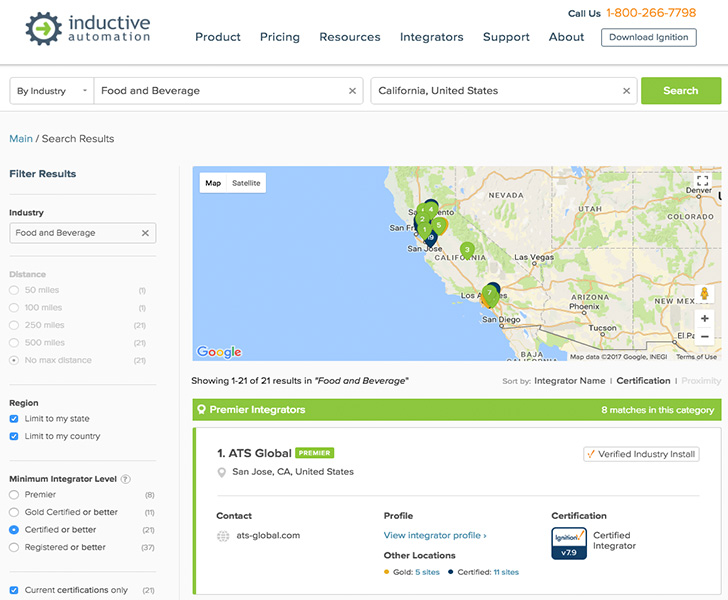In this image, positioned at the top, there is a header displaying the following text: "Inductive Information, Product, Price & Resources Integrators Support." Adjacent to this, there is a button labeled "Download Ignition" and a contact number "Call Us: 1-800-266-7798."

Below the header, there are two prominent boxes. The first one is labeled "By Industry," with a subcategory "Food and Beverage." The second box indicates the location "California, United States." Beneath these, a green "Search" button stands out.

The primary visual element of the image is a Google map displaying the southwestern United States. Numerous green location pins are scattered across California. 

Underneath the map, the text states: "Showing 1 to 21 of 21 results in Food and Beverage - Sort by Integrator Name, Certification." Following this, a green-highlighted section reads: "Premier Integrators - 8 Matches in this category."

The first entry in the list is prominent, detailed as follows: 
"1. ATS Global, San Jose, California, United States."
The text further indicates that this integrator is verified in the food and beverage industry with the status "Installed." Additional actionable options include "Contact: contact@ats-global.com" and a button "View Integrator Profile."